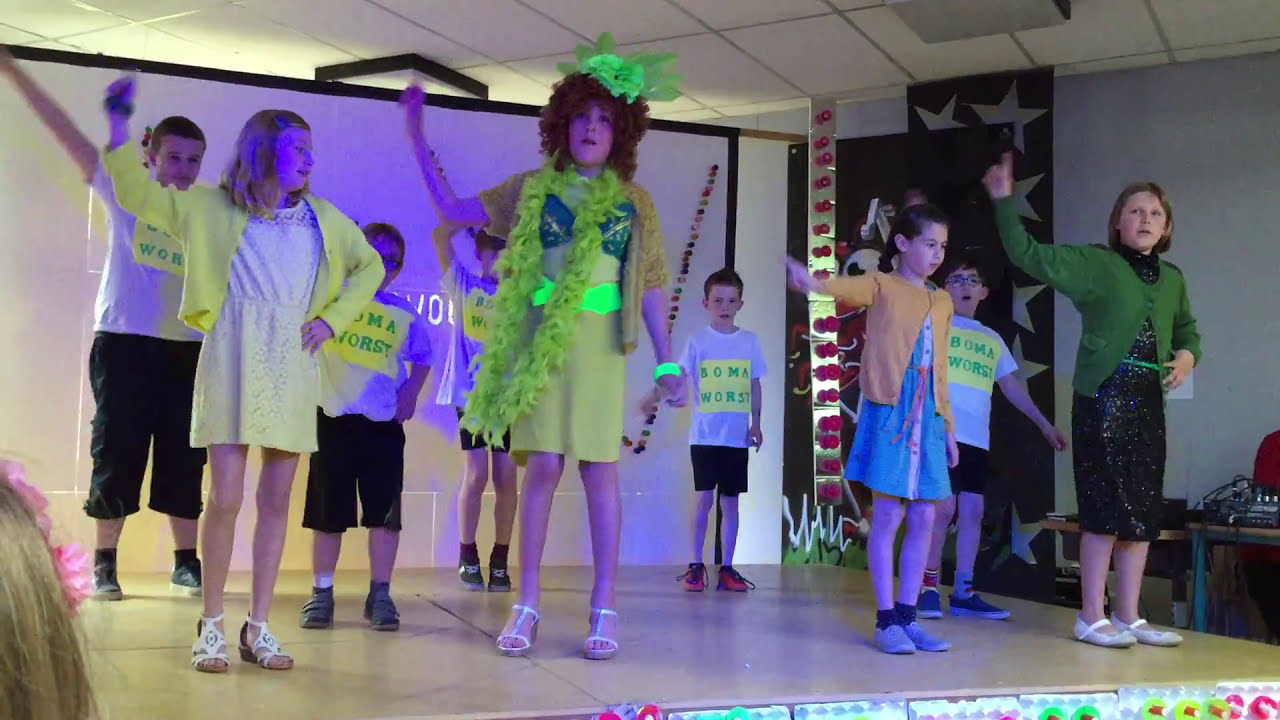The image features a group of children on a small, decorated stage. Positioned in two rows, the front row consists of four girls dressed in vibrant outfits. From left to right: the first girl wears a yellow cardigan and yellow dress, with one hand in the air and the other on her hip. Next to her, a girl wearing a curly ginger wig, a green neon headband, a yellow dress, and a yellow lei, also has one hand raised. To her right, a child in a mustard yellow cardigan and blue dress extends one arm outwards. At the end of the front row stands a girl in a black shiny dress and green cardigan, with short blondish hair, one hand in the air, and the other on her waist.

In the back row, there are five boys, each wearing black shorts and matching blue t-shirts with green or yellow emblems reading "BOMA WORST." These boys have varying arm positions, some raised and some by their sides. On the far left, a boy wears a light shirt and black cargo pants, followed by another boy in a blue shirt and black shorts. Behind them, partially visible, is another child with the same blue t-shirt. To their right, three additional boys are similarly dressed, one of whom wears glasses.

In the background, a whiteboard is visible, along with a wall decorated with posters and large stars. Red lights, stars, and a central blue light contribute to the stage's festive atmosphere. The audience's viewpoint includes the back of a head in the bottom left corner, featuring blonde hair adorned with pink flowers. The children on stage vary in age, appearing to range from approximately six to twelve years old.